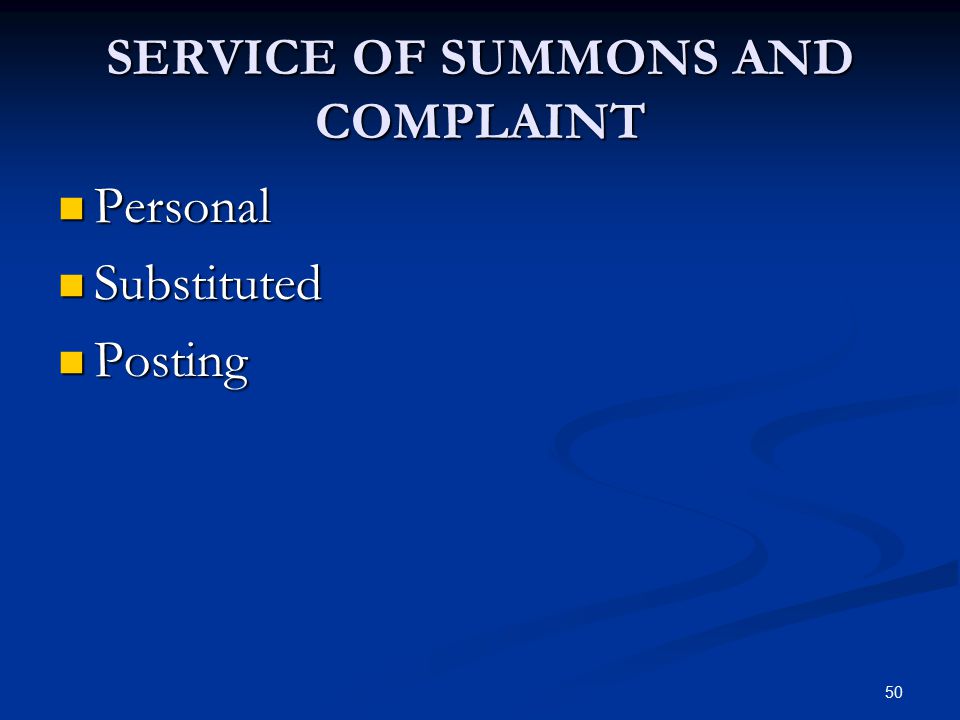In this PowerPoint slide, which features a predominantly dark blue background, the title "Service of Summons and Complaint" is prominently displayed at the top in white text. Below the title, there are three distinct categories listed vertically on the left side of the slide: "Personal," "Substituted," and "Posting." Each category is marked with a yellow square bullet point. A logo that resembles a pair of overlapping S’s, possibly designed to look like a ripple, is situated in the bottom right corner, alongside the slide number "50" in white text. The overall layout and style suggest that this slide is part of a formal presentation, possibly intended for legal or educational purposes, such as a YouTube tutorial, a classroom lecture, or a court instruction.